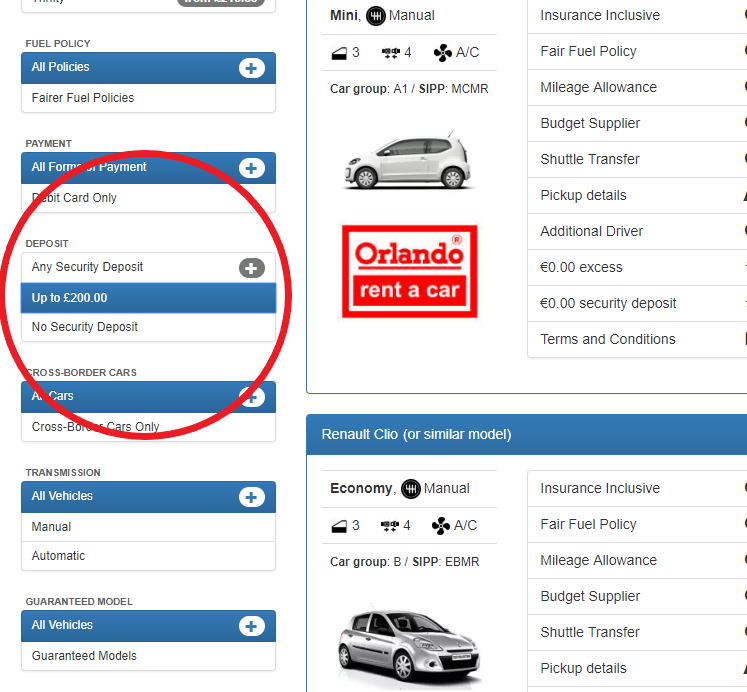### Detailed Caption

In the image, we observe a webpage with a predominantly white background, accentuated by various blue bars that delineate different sections of the page. Scattered among the white and blue areas are bits of red and black text, providing additional details.

On the left-hand side of the page, several headers are visible. The topmost header, "Fuel Policy," is followed by sections like "All Policies" in blue, accompanied by a plus sign, and "Fare Fuel Policies" beneath it. Next, the "Payment" section has subcategories such as "All Format Payments" with a plus, "Debit Card Only," "Deposit," and "Any Security Deposit" with a plus. This section further highlights "Up to 200 Pounds" in blue and "No Security Deposit."

A red circle prominently wraps around the "Payment" and "Deposit" sections. Below this circled area, there is another section labeled "Cross Border Cars," with options like "All Cars" and "Cross Border Cars Only." These three sections are collectively enclosed within a large red circle.

Further down on the left, the "Transmission" section lists "All Vehicles" with a plus, "Manual," and "Automatic." Adjacent to this, the "Guaranteed Model" section includes "All Vehicles" with a plus, followed by "Guaranteed Models."

To the right of the page, an image of a car is displayed within a square box labeled "Orlando Rent a Car." Above the car, various icons are visible: a door icon with the number three, an AC symbol, a manual transmission symbol, and an insurance icon. Additional text surrounding the image lists attributes such as "Insurance," "Inclusive Fare Fuel Policy," "Mileage Allowance," "Budget Supplier," "Shuttle Transfer," "Pickup Details," and "Additional Details," though some of these sections are truncated.

Beneath the car image, the text "Renault Clio" identifies the vehicle model, described further by terms like "Economy," "Three Doors," "Four Seats," "AC," "Car Group B," and coded identifiers "SIP, EMB, EBMR." Another silver car image is situated below this description.

In summary, the webpage appears to focus primarily on the left side, emphasizing the circled sections that prompt user interaction.